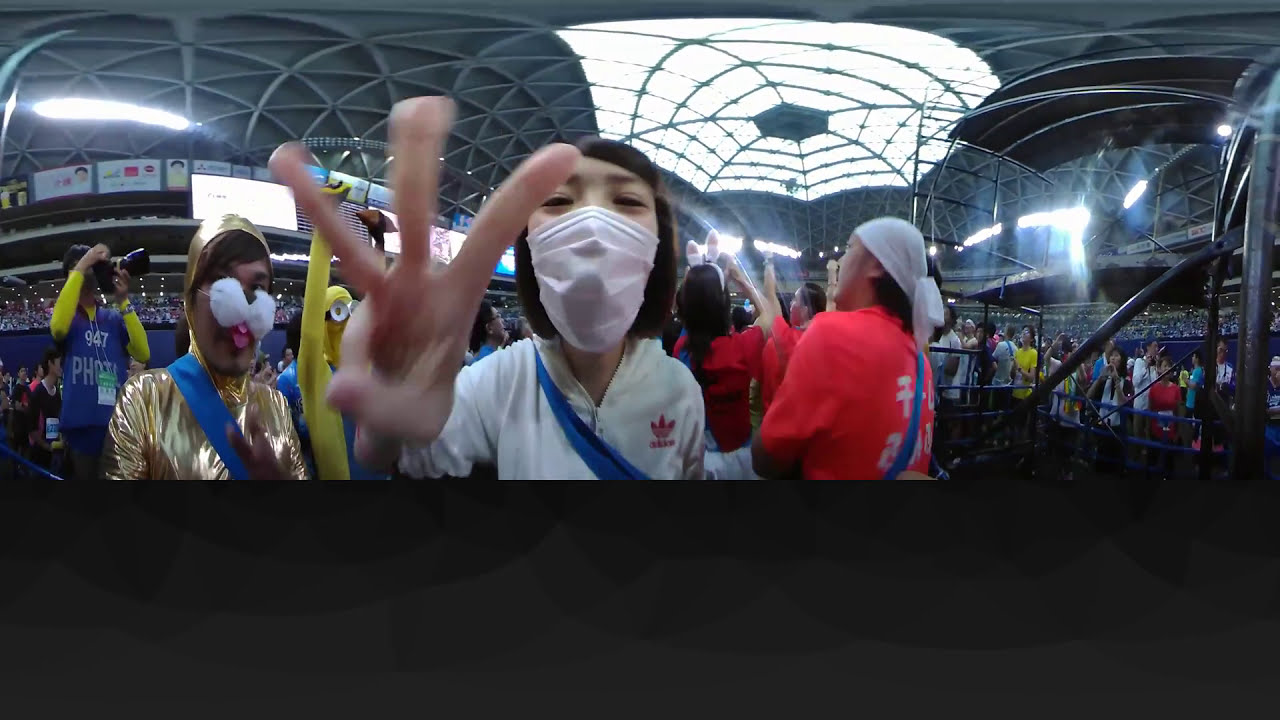In a bustling, well-lit stadium filled with spectators, a young Asian girl, approximately 12 years old, stands in the foreground, beaming behind her white surgical mask. She confidently holds up three fingers to the camera, hinting at her excitement. Her black hair falls to her shoulders, and she's dressed in a white Adidas sweatshirt with a blue strap from her book bag across her shoulder. To her left stands a boy in an eye-catching gold suit, reminiscent of an alien costume, complete with a white furry nose and tongue sticking out like a cat. On her right, another man is seen in a red shirt with white lettering and a white bandana, also sporting a blue strap around his shoulder. The scene unfolds in an auditorium, likely somewhere in Asia, with a distinctive scalloped roof and stands filled with spectators in the background.